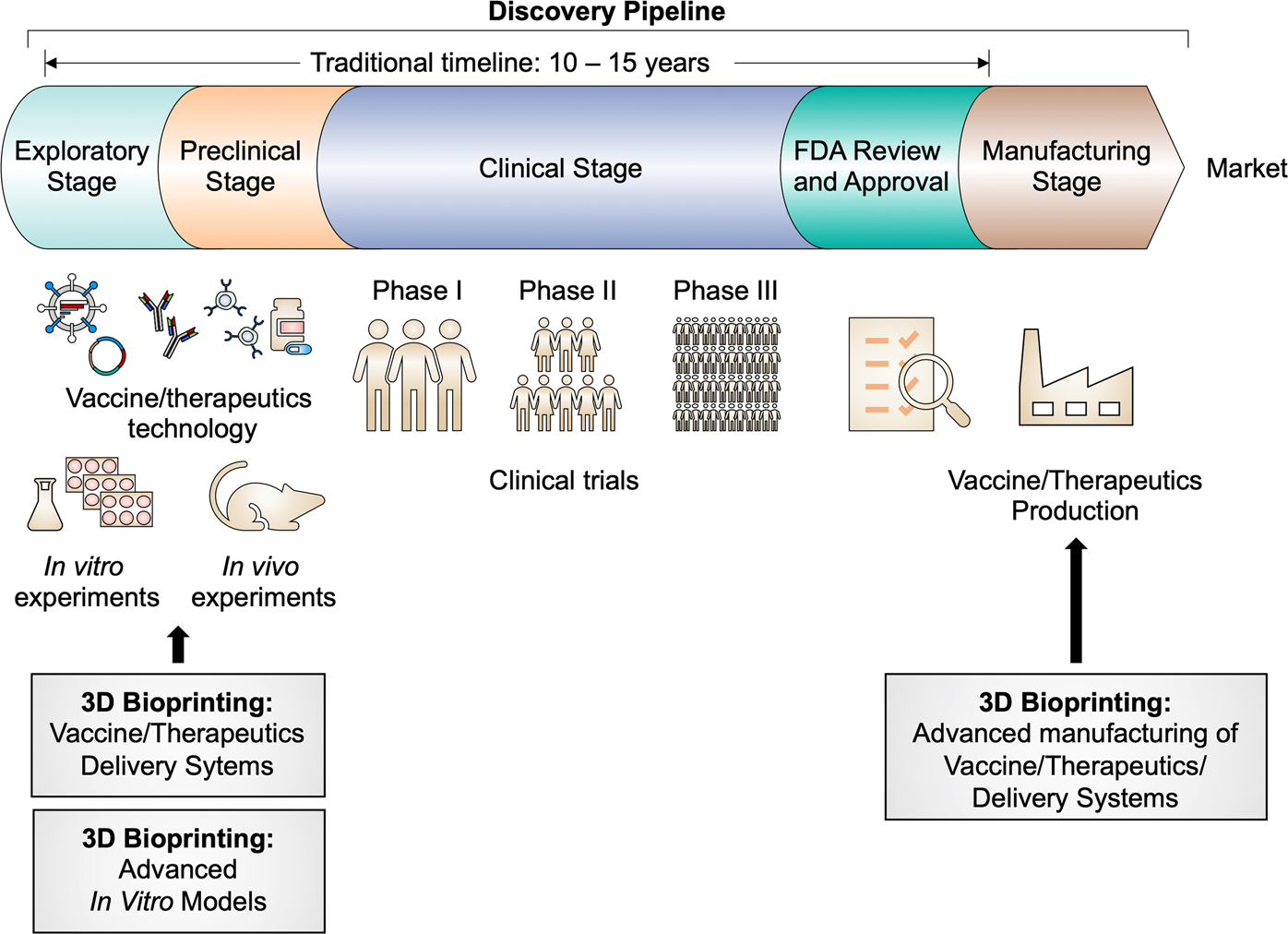This illustration depicts the 3D bioprinting process for vaccine therapeutics. At the top, a detailed "discovery pipeline" graph outlines a traditional 10-15 year timeline, which includes the stages: exploratory, preclinical, clinical, FDA review and approval, manufacturing, and finally, market entry. Below this timeline, various diagrams further break down the process. These include representations of vaccine therapeutic technology, such as vials, pills, and racks for in vitro experiments, as well as different phases of clinical trials. Phase 1 is shown with 3 people, Phase 2 with 8 people, and Phase 3 with an even larger group. Also depicted is a paper with a magnifying glass, symbolizing detailed analysis and documentation. At the bottom of the illustration, three squares highlight key components related to 3D bioprinting: "3D Bioprinting," "Vaccine Therapeutic Delivery Systems," and "Advanced In Vitro Models," along with "Advanced Manufacturing of Vaccine Therapeutics Delivery Systems." The color scheme includes white, tan, light blue, pink or peach, light purple, and teal.